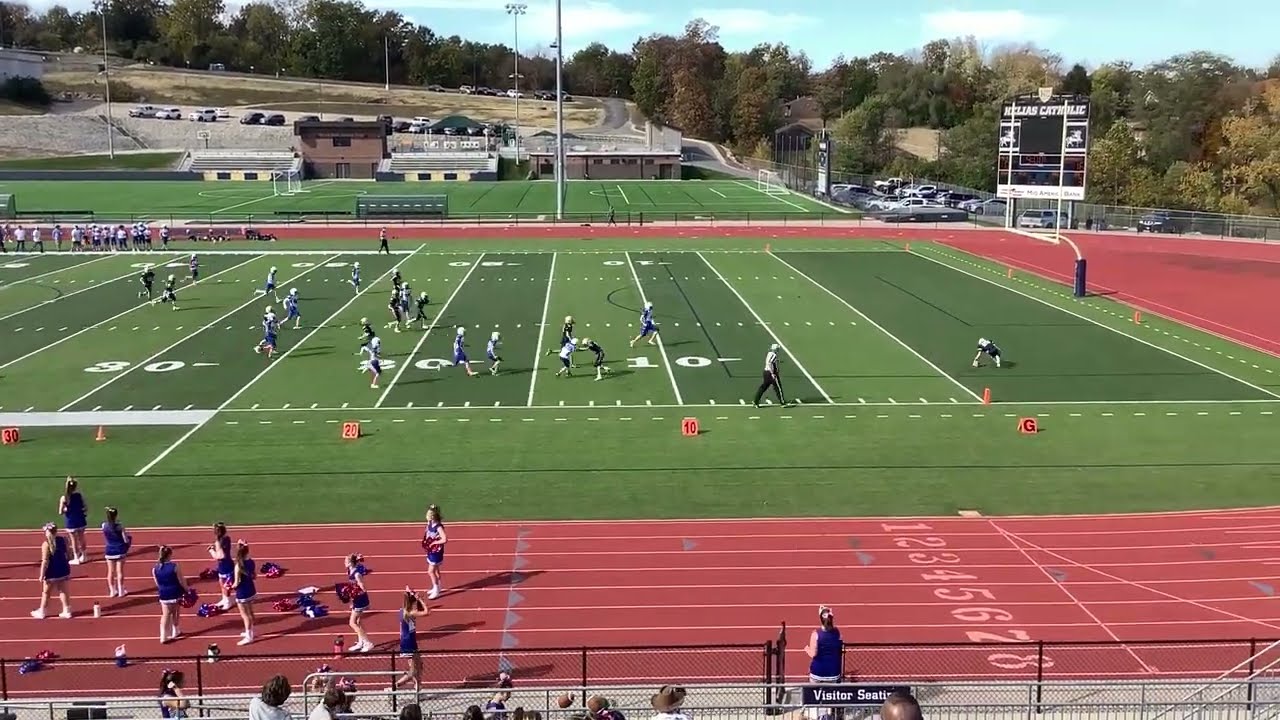The photo depicts a high school football practice taking place on a well-maintained football field. Players dressed in dark jerseys can be seen running towards the end zone, with the 10, 20, and 30-yard line markers clearly visible. A referee is positioned on the sideline, overseeing the practice.

In the foreground, a group of cheerleaders dressed in blue uniforms and holding pom-poms are spread out on a red track that encircles the green football field. Some cheerleaders are attentively watching the practice, while others are facing different directions. The track area also features audience bleachers, which appear to be mostly empty with a few spectators visible.

On the right side near the bottom of the image, a sign indicates "visitor seating," and behind the goalpost, another sign reads "Kellers Catholic," identifying the school. In the distant background, there are more fields, including a soccer field, as well as a parking area with cars, streetlights, and an expanse of trees. The scene is set under a blue sky with scattered clouds, creating a vibrant and active sports environment.